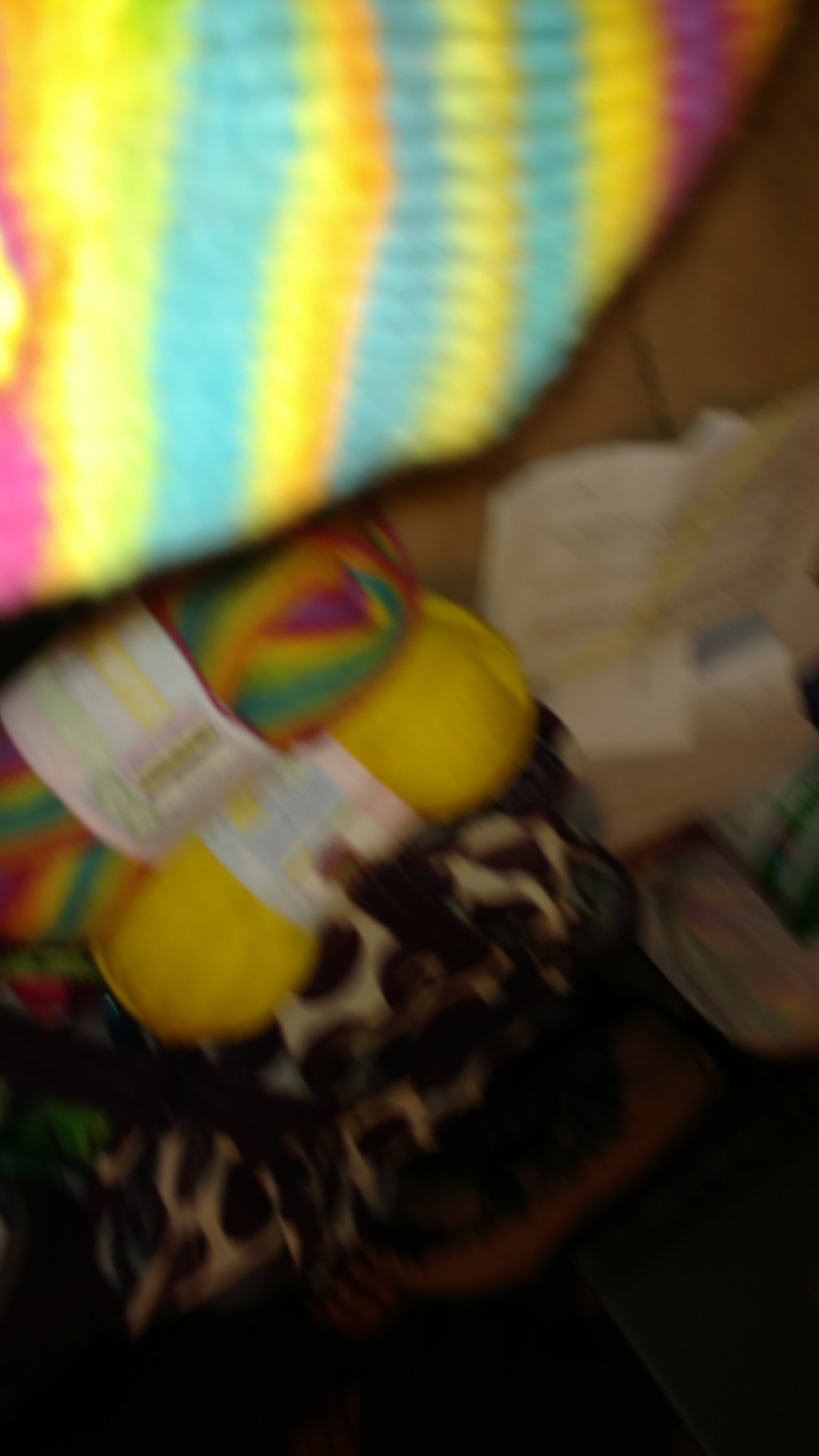The image depicts a slightly blurred scene featuring a colorful, striped blanket draped horizontally from right to left. The blanket displays an array of colors in the following sequence: pink, yellow, purple, yellow, light blue, yellow, light blue, darkish yellow, light blue, bright yellow, and a lighter pink. Beneath the blanket, there are skeins of yarn in varying colors, including yellow and a multicolored one, wrapped in white paper packaging. This yarn appears to be placed on a dark-colored material, potentially a piece of cloth with black, brown, and beige tones. Additionally, there are a couple of circular objects on the light brown wooden floor—one orange with a white center and the other red, yellow, and green striped. To the right, some white sheets of paper or possible receipts with indistinguishable black text are present, completing the scene.